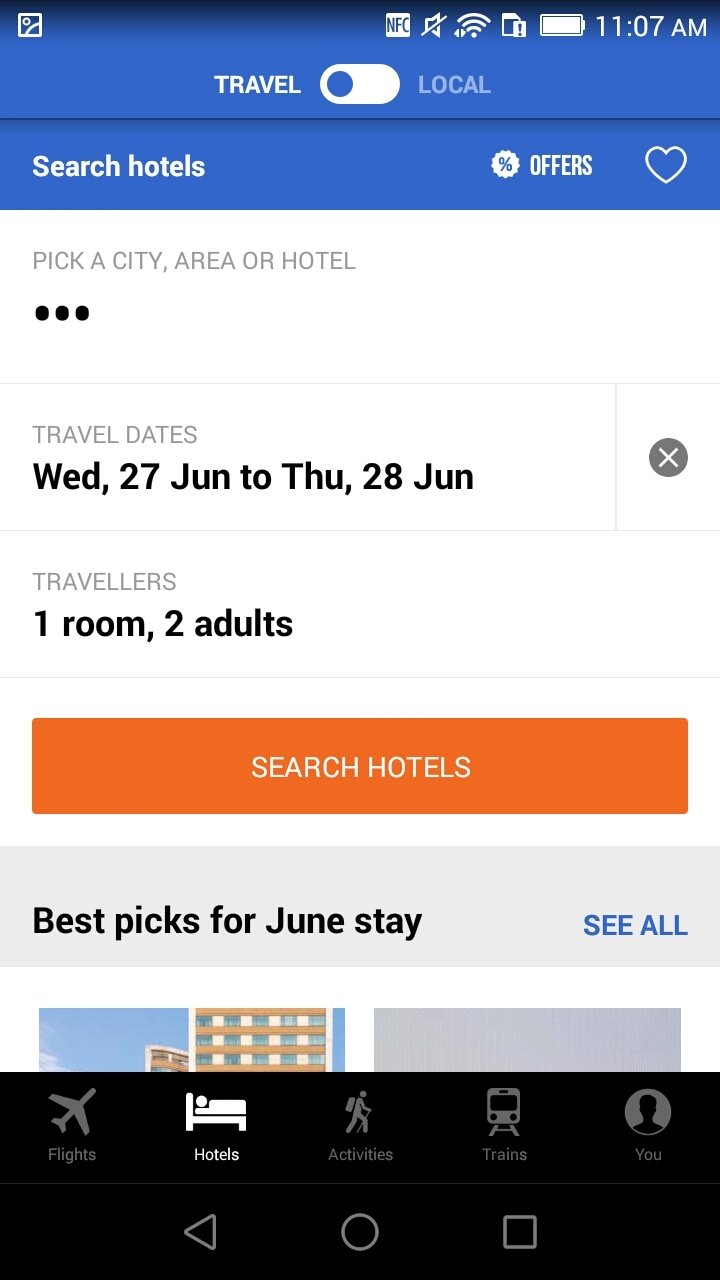This is a detailed screenshot from a travel mobile app, featuring a blue header at the top. The header includes two toggles labeled "Travel" and "Local," with the "Travel" option currently selected. Above the header, the status bar displays several icons on the right side: NFC, mute, battery, and the time (11:07 AM).

Below the toggles in the header, there are two sections: one on the left stating "Search hotels" and another on the right showing "Percent offers" accompanied by a heart emoji. Immediately beneath the blue header, the page background turns white, presenting a search input area with the prompt "Pick a city, area, or hotel" and three black dots indicative of a carousel or multiple tabs.

Further down, there's a section summarizing travel dates, displaying "Wednesday 27 June to Thursday 28 June." Following this, another row provides information about the travelers, specifying "1 room, 2 adults." Below these details is an eye-catching orange "Search Hotels" button.

Continuing down the page, a line announces "Best picks for June stay" alongside two partially visible photographs, indicating curated options or recommendations. A "See all" link is positioned to the right of this section for expanded viewing.

At the bottom, the footer is colored black and features five icons in a row. These icons represent different categories within the app: "Flights" (an airplane icon), "Hotels" (a bed with a person laying down), "Activities" (a hiker with a backpack), "Trains" (a train head-on), and "You" (a silhouette of a person's head).